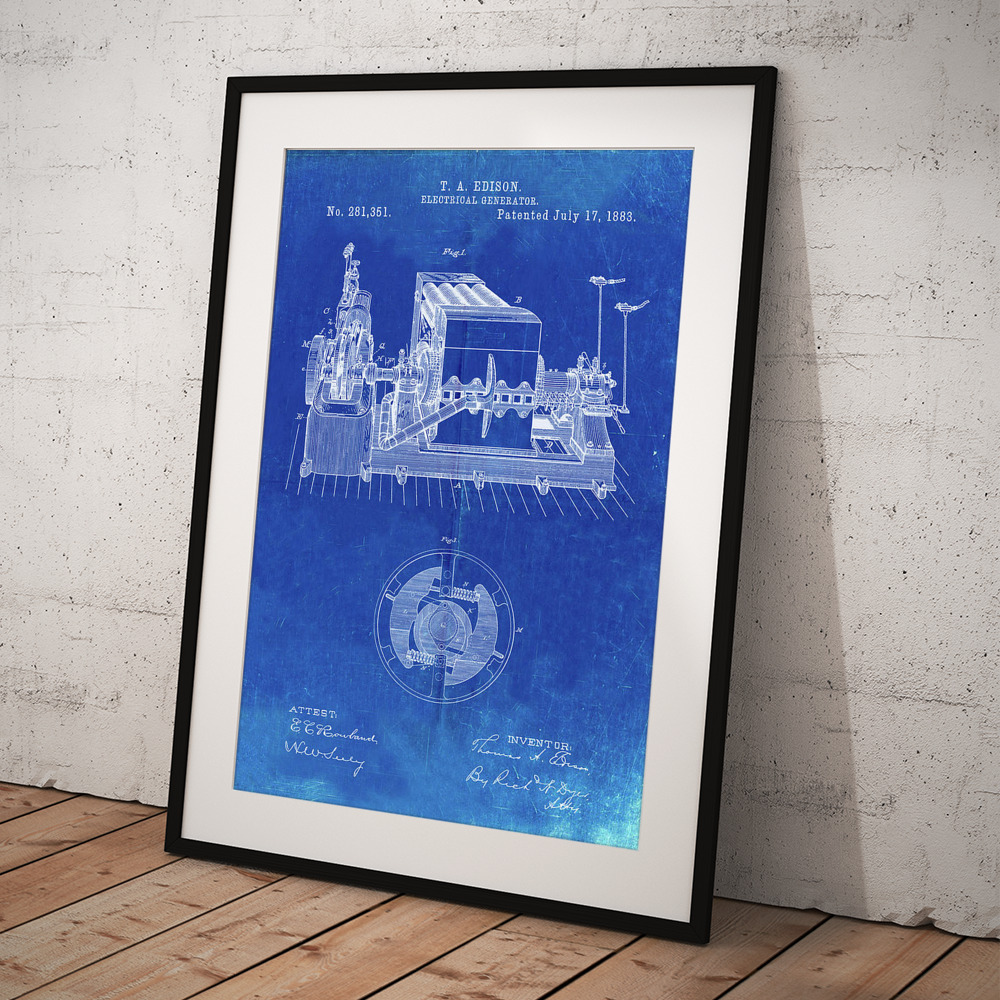A black-framed blueprint rests against a white wall on a wooden floor. The blueprint paper is a deep blue adorned with intricate white detailing. At the top, it boldly states, "T.A. Edison, Electrical Generator," with the specifics "Number 281,351" on the left and "Patented July 17, 1883" on the right. The centerpiece of the blueprint is a detailed diagram of what appears to be a generator, featuring a large rectangular box with four tubes running across the top and additional mechanisms below. The sides of the box are open, revealing further machinery and components attached that extend to the right. Tall, slender pipes or rods rise on either side of the box, and on the lower left of the generator, intricate gears are visible. Beneath this, a round diagram displays more complex mechanisms. Cursive signatures mark both the lower left and lower right corners, identifying the inventor, Thomas Edison, and another individual, likely attesting to the patent's authenticity. The black frame includes a white border, enhancing the blueprint's historical and technical significance.